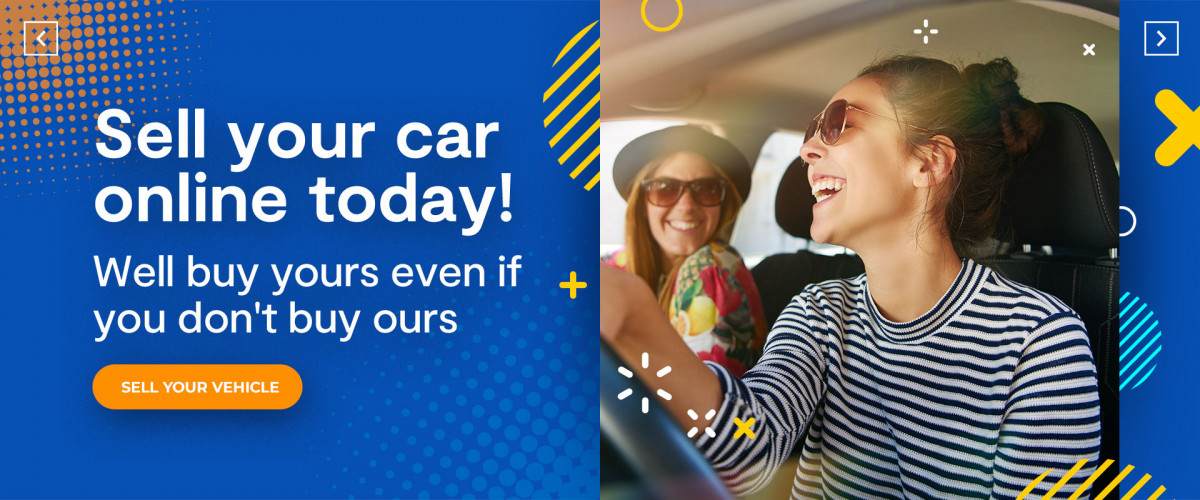A vibrant digital advertisement dominates the scene, with a long rectangular shape suggesting dimensions of approximately 30 by 70, providing a wide yet slim visual. The left side of the ad features a rich blue background with bold white text that exclaims, "Sell your car online today!" followed by the tagline, "We'll buy yours even if you don't buy ours." Below this text, an inviting orange button stands out, emblazoned with "Sell Your Vehicle" in white font.

Adding to the ad's playful and engaging design, the top left corner showcases a cluster of small orange dots, which gather in a whimsical pattern. The background is further adorned with a series of flowing yellow and blue lines, contributing a sense of dynamism and personality.

Transitioning to the right side of the ad, the blue background continues, complemented in the upper right corner by a stylized box with an arrow pointing to the right, driving the viewer’s attention towards the adjacent image. This image features a joyful scene inside a car: two women sharing a lively moment. The driver, a young woman with her brown hair tied up in a knot, sports a black and white striped long-sleeve shirt and sunglasses. She is laughing heartily. Next to her, seated on the left, is an older woman wearing a black hat and a vibrant shirt with pink, yellow, and green stripes. The serene expression on her face suggests she might be the driver’s mother, adding a warm, familial touch to the advertisement.